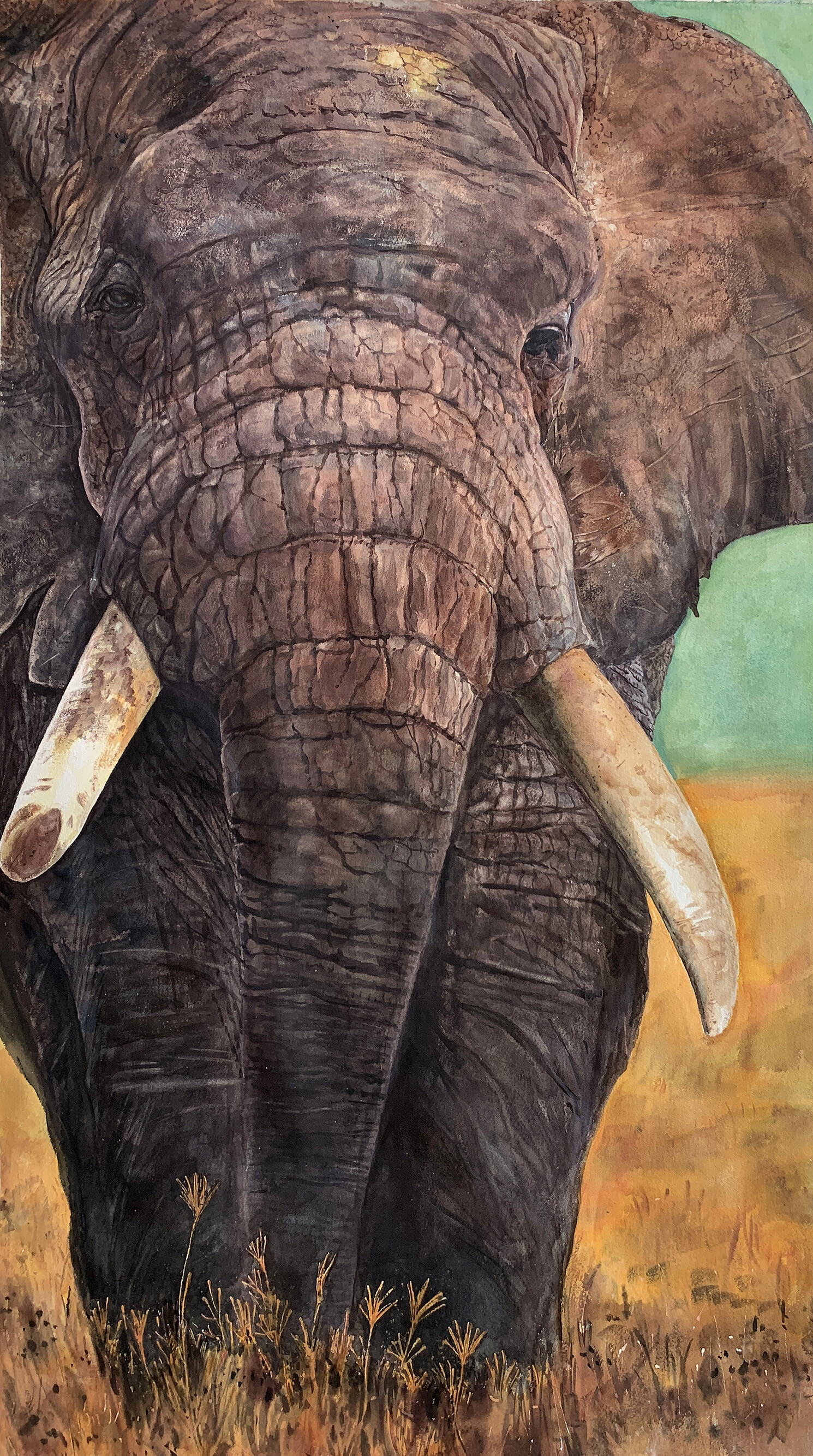This image is a detailed, vertically oriented painting of an imposing, older elephant set against a backdrop that's both wild and desolate. The scene is dominated by earthy hues, with the background characterized by a predominantly tan, African grass field that looks parched and dead. The foreground and background blend into a rough, brown area cluttered with weeds that reach up to the elephant's ankles. The elephant's gigantic form takes center stage, so large that its full body and ears can't be entirely seen within the frame.

The portrait focuses primarily on the elephant's massive snout and tusks. Its tusks are a striking combination of yellowish-tan and white, aged and worn, with one potentially appearing broken. The elephant's weathered gray skin varies in tone from light to dark, particularly darker toward the bottom of its powerful legs. The creature's black eyes and large ears contribute to its ancient and majestic demeanor. The horizon and sky, only slightly discernible, are painted in a teal color visible mainly on the upper right corner and middle right side of the picture, just beneath the thick presence of the elephant, which is slightly off-center to the left.